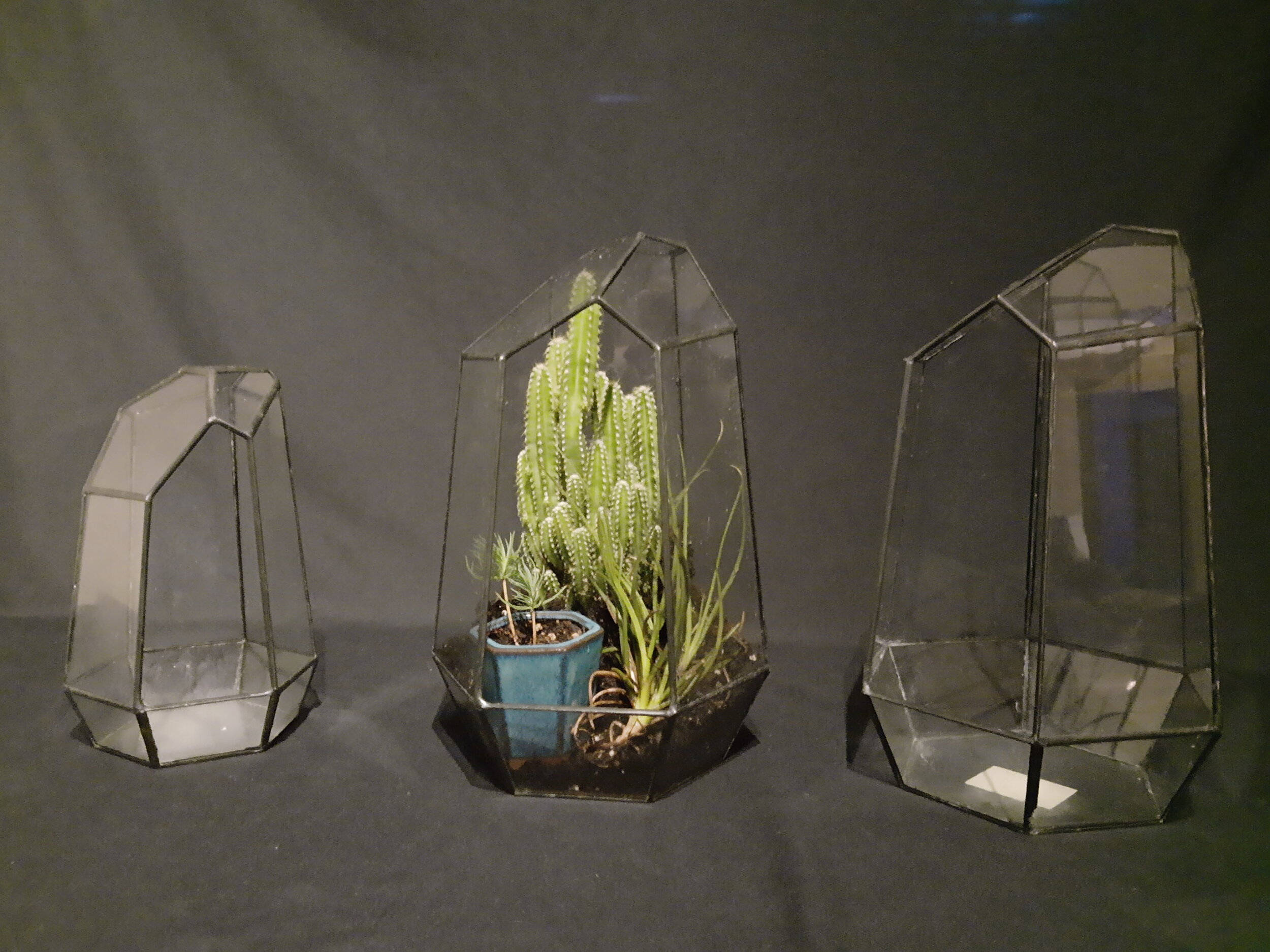The image showcases a set of three tabletop terrariums, each varying in size and arranged on a table covered with a gray cloth. The terrariums are clear and have black-lined edges, resembling crystalline structures with their odd angles and sharp lines. From left to right, the terrariums are placed in ascending order of size. The smallest terrarium on the left and the largest on the right are both empty, highlighting their intricate glasswork. The middle terrarium, slightly smaller than the largest one, contains an assortment of plants. Inside it, a tall cactus reaches toward the top, while a blue pot houses a small, tree-like plant. Additionally, another unidentified plant resembling onions is planted directly in the soil. The overall color palette of the image includes shades of black, gray, green, blue, and brown, with the shiny gray background reflecting parts of the scene to add depth. This detailed arrangement is likely to intrigue plant enthusiasts and those interested in home decor or DIY projects.